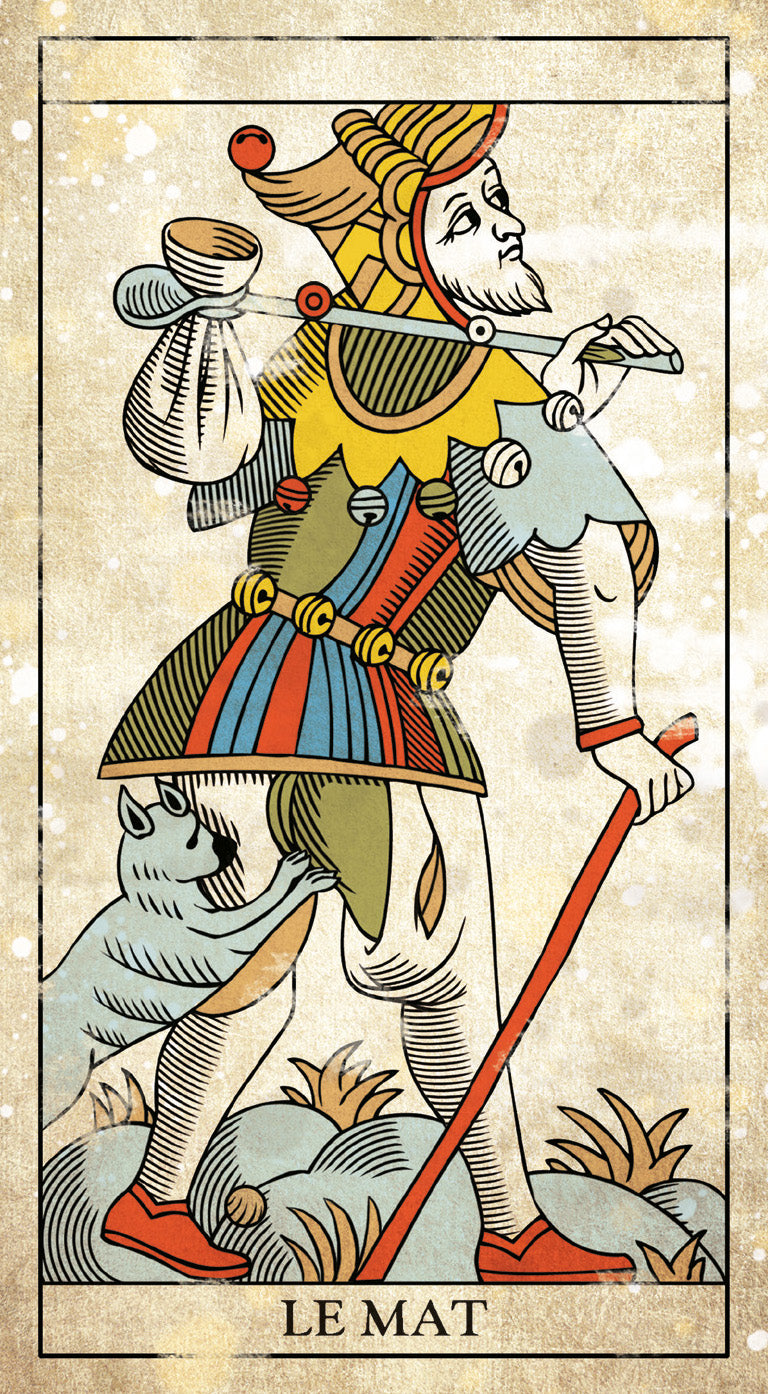This detailed illustration appears to be a vintage tarot card, specifically of "Le Mat" or "The Fool", evident from the text at the bottom of the card. The artwork, which exudes a weathered and aged texture, features medieval-style, flat, and hatched lines, immersing the viewer in an antiquated feel. The card’s dimensions are portrait-oriented, with an inner and outer border framing the central image, both of which contribute to its classic appearance.

Dominating the card's center is a richly-dressed, jester-like figure, adorned with a multicolored outfit that includes red and blue patterns, a yellow collar, and a pointed, bell-adorned neckpiece reminiscent of a traditional joker’s attire. He also sports a distinctive hat with a red bell at its peak and a scraggly beard, enhancing his whimsical look. 

The figure’s posture suggests motion; he carries a hobo sack—an old-fashioned stick with a small white bag tied to its end—slung over his right shoulder, while his left hand grips a red walking stick. His eyes gaze upwards, adding a sense of wanderlust or contemplation to his demeanor. 

Behind him, a small, blue dog paws or bites at his back leg or buttock, injecting a sense of motion and playfulness into the scene. The ground at his feet is strewn with white rocks and brownish grass, encapsulating the earthy textures typical of ancient tarots.

Overall, this image faithfully represents "The Fool" from a traditional tarot deck, blending medieval aesthetics with evocative, illustrative storytelling.